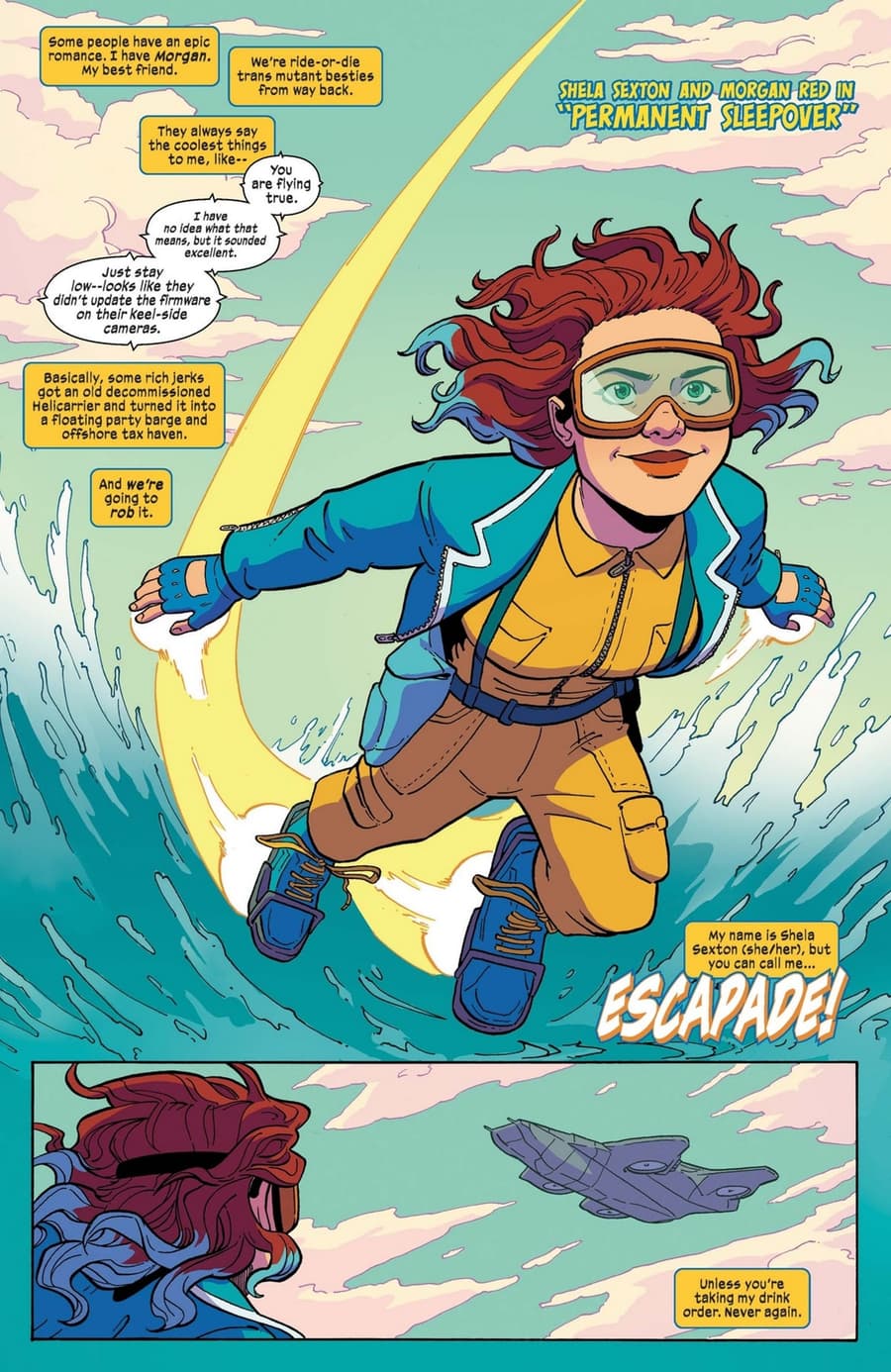The comic book illustration features a dynamic scene with a light blue background and a red-haired superhero named Selah Sexton, also known as Escapade. She is depicted mid-flight, diving into the water with wild red hair accented by blue tips. Escapade is wearing a blue coat jacket over a distinctive yellow zip-up bodysuit, complete with large pockets along the thighs and blue boots with yellow laces. The scene suggests she's either floating or diving into the water, as indicated by a big wave beneath her. The caption prominently displays the title "Selah Sexton and Morgan Red in Permanent Sleepover", with the word "ESCAPADE!" in large, striking letters. In the foreground, small dialogue bubbles can be seen, though the text is difficult to read. Another inset panel shows Escapade underwater, looking up at what appears to be a futuristic submarine or possibly a plane, suggesting she might have jumped from it. Overall, the colors are vibrant, with a combination of blue, yellow, and orange, highlighting her adventurous and bold character.